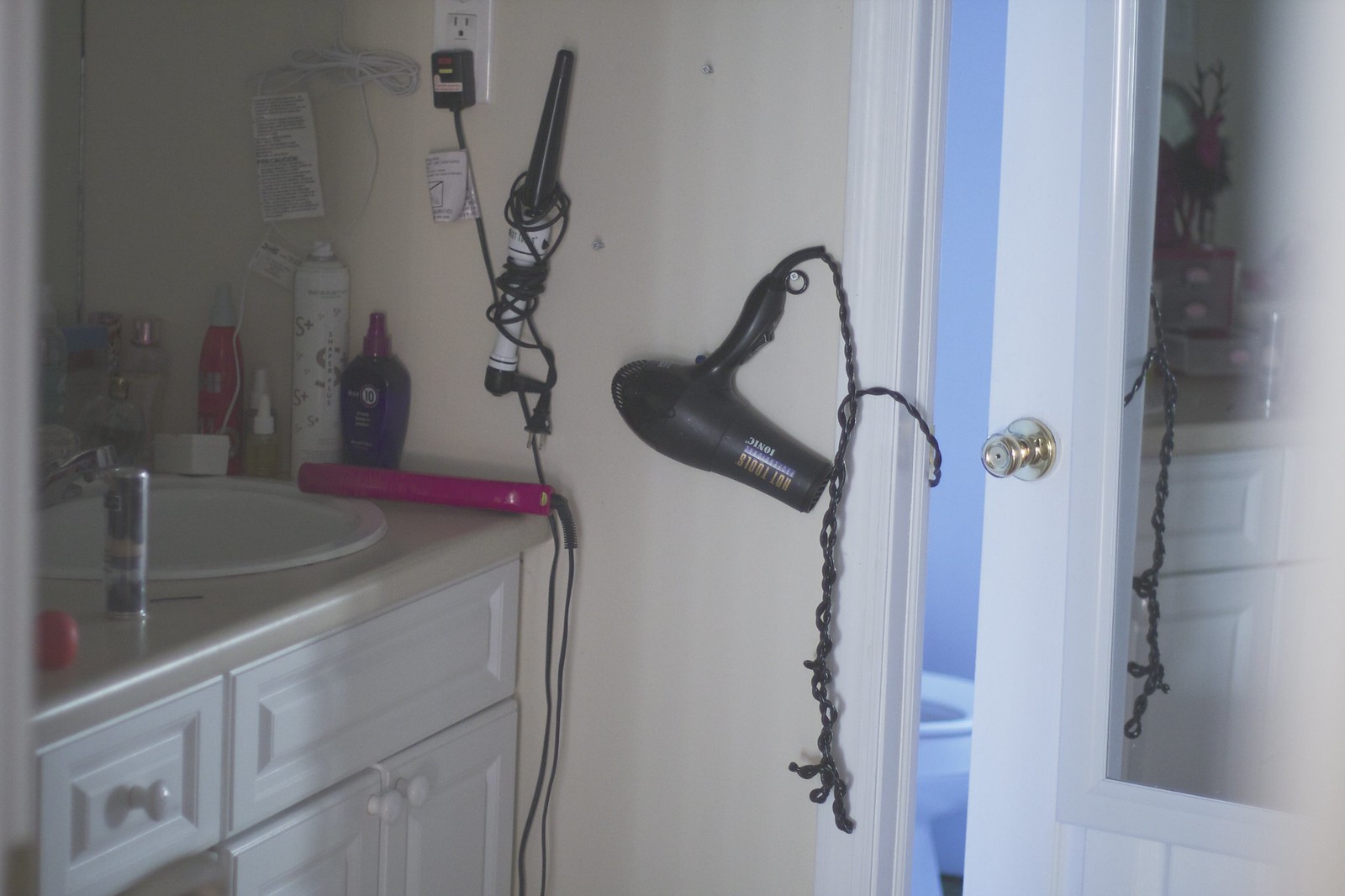The image depicts a somewhat cluttered bathroom with an ivory-painted wall and a separate, slightly ajar door leading to a toilet room. The door features a mirror and reveals a glimpse of a blue wall and toilet inside. To the left of the door, a heavily tangled cord is connected to a black hair dryer hanging on a hook. The bathroom's white sink is mounted on a cream-colored Formica countertop, complemented by white drawers and cabinets below. On the counter, a pink hair straightener with its cord trailing to the floor is plugged into an outlet near a curling iron, which also hangs on the wall with its cord wrapped around it. Various bottles, including perfumes and hair care products like Miracle 10 in a distinctive blue bottle with a light purple lid, are scattered around the sink area, adding to the disorganized appearance. There are clear storage cabinets visible in the mirror's reflection, suggesting more storage on the opposite side of the room.